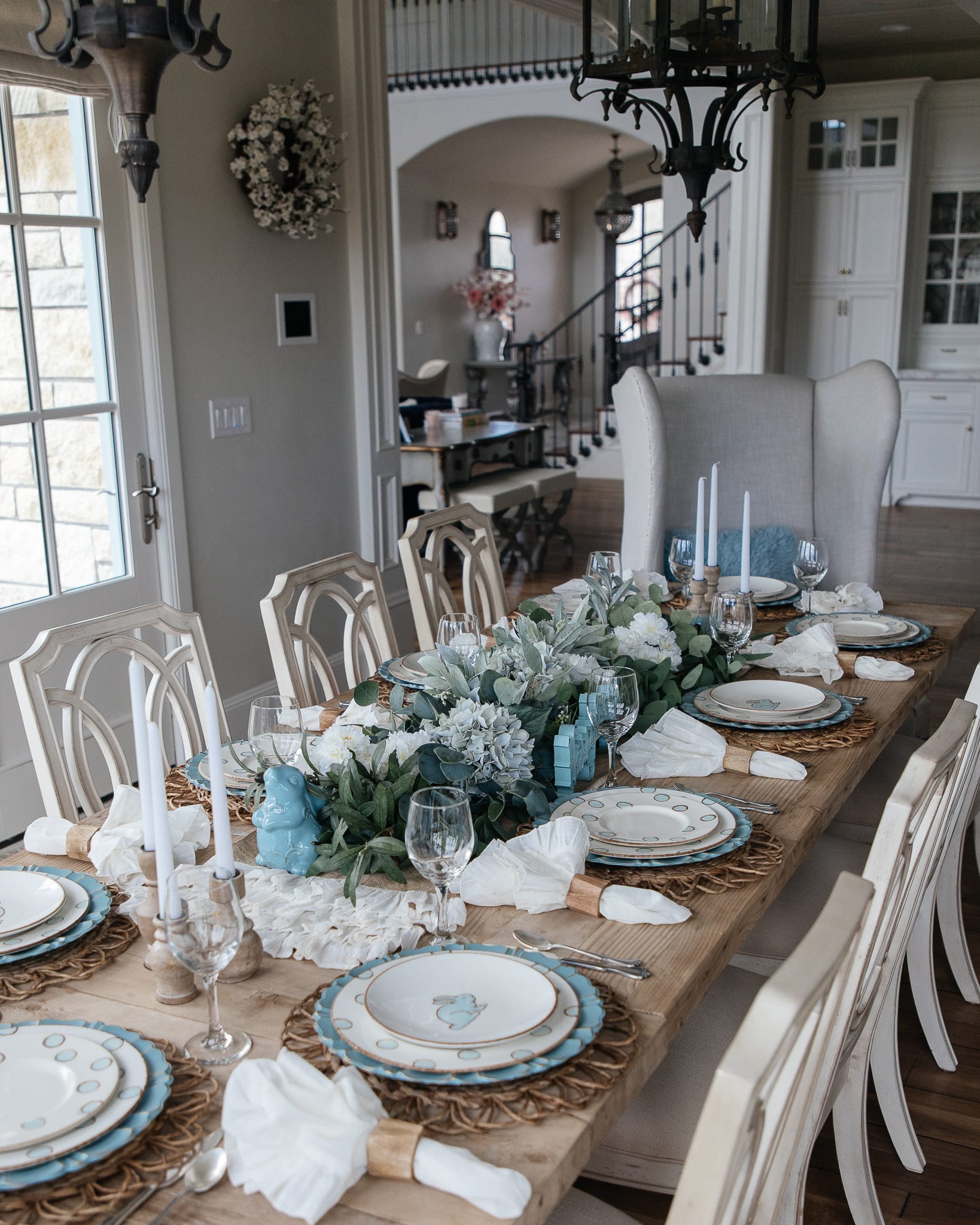This vertically aligned image captures the elegant interior of a predominantly white dining room with a sophisticated table setup. The majority of the home is white, including the walls, ceilings, and the white chairs that encircle a large, light brown wooden rectangular dining table. The table is neatly set with wicker placemats and stacked plates at each setting. Each stack consists of a large blue plate at the bottom, a medium white plate with spaced large blue polka dots in the middle, and a smaller top plate featuring a blue rabbit partially visible on its right side. 

In addition to the plates, the table also boasts white napkins with rings, unfilled wine goblets, silverware, and white candlesticks at each end. The centerpiece includes a beautiful assortment of bluish-white flowers and succulents, enhancing the table's refined appearance. 

In the background, there is a staircase leading to the next level, a chandelier hanging from the ceiling, and a visible front door with windows showing a brick wall outside. A large white vase with flowers is placed on a shelf near the door, adding to the room's decor. The walls are a soft tan color, accented by white woodwork, and additional details include cabinetry on the upper right and a wreath on the left wall. The overall ambiance exudes elegance and charm, with the cohesive colors of white and light blue harmonizing beautifully.